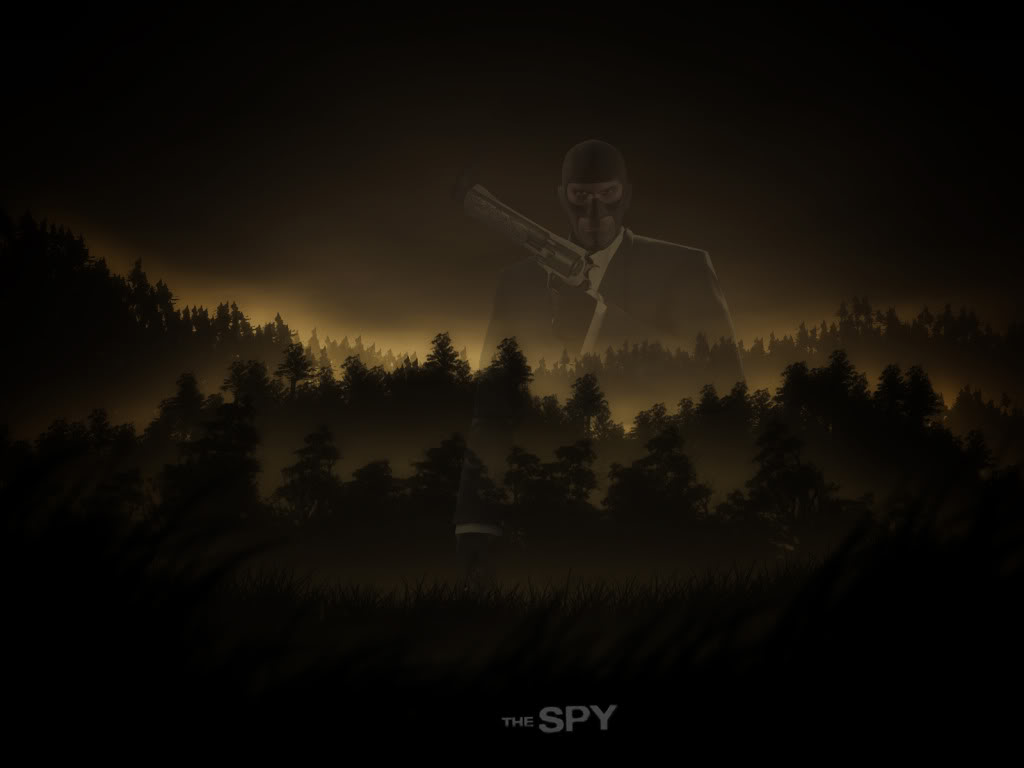In this dark, eerie image, a shadowy forest forms the backdrop, with a blend of indistinguishable pine trees shrouded in near-black darkness. The sky transitions from an ominous black at the top to shades of gray, finally merging into a faint, orange-yellow mist near the horizon. The foreground grows progressively darker, casting an almost sinister ambiance.

At the center of the image, standing against the obscured tree line, is the ghostly figure of a man. He is dressed in a black suit jacket over a white shirt, with black gloves that further accentuate his menacing appearance. His face is partially obscured by a mask that covers his head and nose, leaving his piercing eyes and mouth exposed. His intense, unsettling gaze seems to penetrate the viewer. In his left hand, he clutches a large handgun, pointed towards the upper left corner of the frame, adding to his threatening aura. The ambiguity of his blurred form only heightens the sense of dread.

At the bottom of the image, the gray words "THE SPY" are prominently displayed, with "SPY" in all caps and larger than "THE," grounding the mysterious figure in an enigmatic narrative of espionage and covert operations.